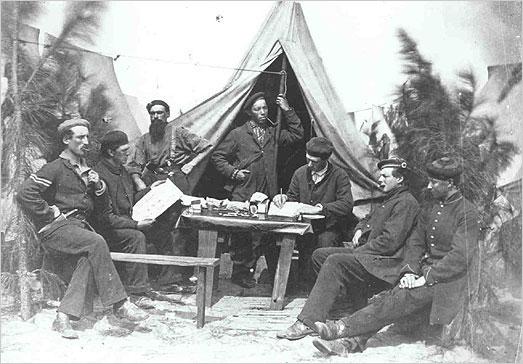This antique black and white photograph captures a group of seven men gathered at a campsite, sitting around a rough-hewn wooden table. The backdrop features a pitched canvas tent, its flaps open, supported by a single pole. The tent is surrounded by small pine trees, indicative of an outdoor setting, with a blown-out white sky adding an atmospheric element.

The men are dressed in varied uniforms, hinting at possible military affiliation, with some showing stripes akin to sergeant insignia. All of them don flat hats, and their attire includes long pants and waist-length jackets. On the left, one man, possibly a sailor given his attire and knife sheath, sits on a makeshift bench, smoking a pipe with his hand on his hip and legs crossed. Beside him is another man, dressed in all black, engrossed in examining a large paper. 

Behind them, a man with a long beard, wearing pants, suspenders, and a long-sleeved shirt, stands with his hand resting on his hip. Standing at the tent’s entrance, a younger man in a long dark coat, parade-style hat, and pipe in mouth holds onto the tent pole with one hand, his other hand in his coat pocket. At the table, which is cluttered with various documents, another young man diligently writes on a piece of paper. Additional figures can be seen sitting to the side, contributing to a busy but structured scene that suggests a meeting or briefing in a military camp from the early 1900s.